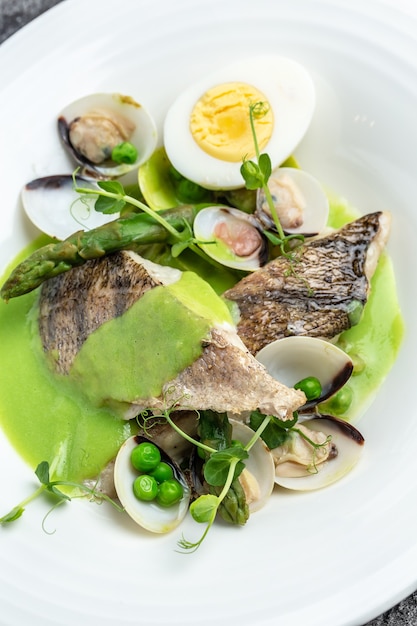This is a close-up, overhead photograph of a meticulously composed lunch plate, centered on a white, shallow bowl. At the heart of the arrangement are two pieces of grilled white fish, each displaying black grill marks and a nice tan color. These pieces are positioned at angles to each other, with one partially covering the other. Both pieces rest in a vibrant green sauce that is spread throughout the base of the dish.

Around the fish, several opened oyster shells, creamy in hue with black accents, contribute to the plate's intricate presentation. One of these shells contains four green peas, which adds a subtle pop of color. More green elements, including a few sprigs of watercress and a single asparagus spear, enhance the dish's freshness. At the top right corner of the plate, half of a deviled egg with a bright yellow yolk stands out prominently amongst the seafood.

This artful arrangement is displayed on a white plate with a glossy sheen, which is set against a sophisticated marble countertop, characterized by gray and black veining. The overall composition not only reflects culinary expertise but also an aesthetic harmony, making the dish visually appealing.